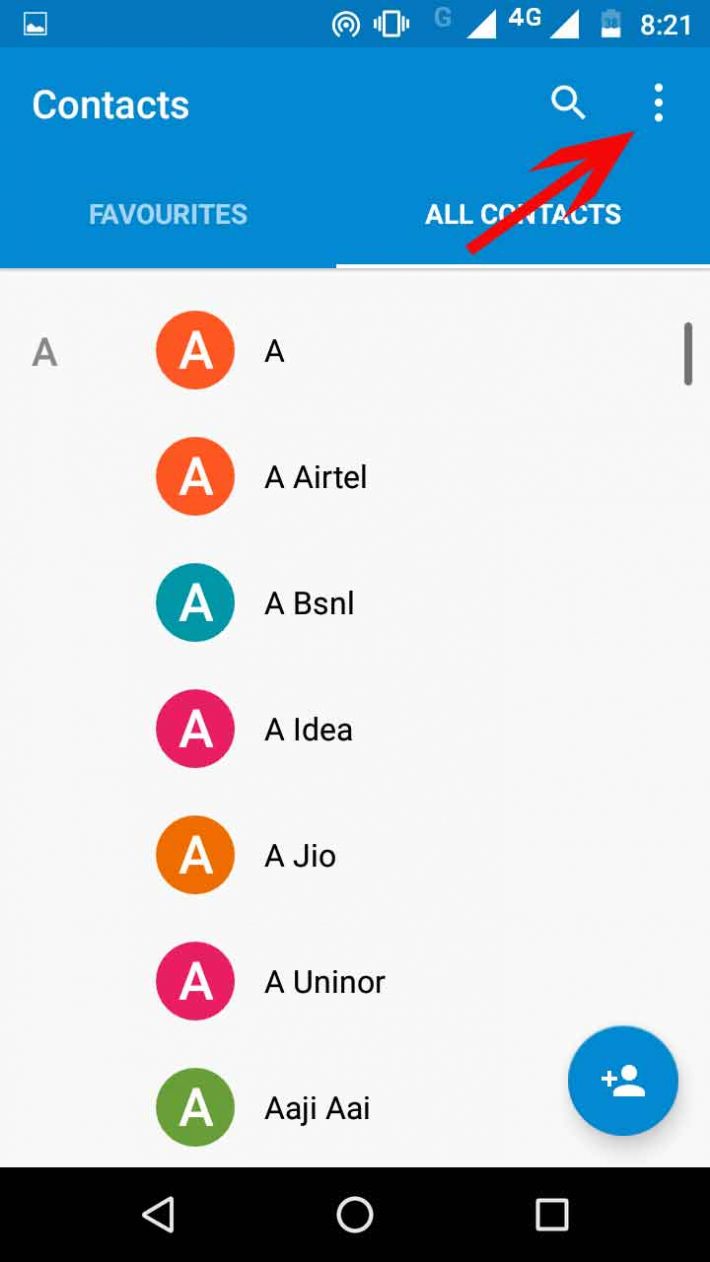This image features a detailed screenshot of a smartphone's contacts screen, possibly from an Android device. Dominating the top of the screen is a blue banner, adorned with various status icons such as Wi-Fi signal, time, and battery life. In the upper left corner, an ambiguous icon—potentially related to the device's orientation (landscape or portrait mode)—is visible.

The blue banner prominently displays the text "Context" and includes tabs for "Favorites" and "All Contacts." Adjacent to these is a search magnifying glass icon. In the far right corner of the banner, three vertical dots represent the settings menu, highlighted by a red arrow pointing toward them for emphasis.

Below the banner is the main contacts list, currently filtered to show entries beginning with the letter "A." On the bottom right of this list, there's a small blue circle featuring an account icon with a plus sign, indicating the option to add new contacts.

At the very bottom of the screen, a black navigation bar houses three essential icons: a left-pointing triangle for the back function, a circle for the home function, and a square for the multitasking view, further suggesting that this is an Android device. Overall, this image meticulously captures the typical layout and features commonly found on an Android contacts screen.